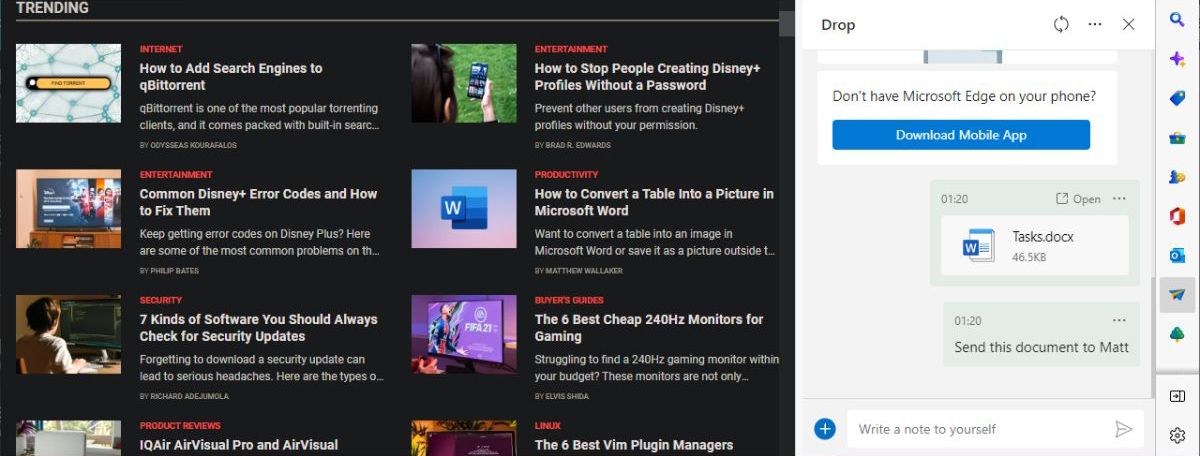A detailed caption for an image based on the provided description:

The image displays a side-by-side view of two screens. 

The left screen showcases a web page with a dark grey background. It features a "TRENDING" header in white at the top left, followed by a thin, light grey dividing line. Below this, a series of articles are listed in a structured format. Each article includes a rectangular thumbnail image, a red category label in all caps, a white title in large text, a brief description in smaller white text, and the author's name in light grey text. The articles are organized in two columns:
- **INTERNET:** "How to Add Search Engines to Qubit Torrent" – Qubit Torrent is one of the most popular torrenting clients, and it comes packed with built-in search... by Odiseas Kixarofolos.
- **ENTERTAINMENT:** "How to Stop People Creating Disney Plus Profiles Without a Password" – Prevent other users from creating Disney Plus profiles without your permission, by Brad R. Edwards.
- **ENTERTAINMENT:** "Common Disney Plus Error Codes and How to Fix Them" – Keep getting error codes on Disney Plus? Here are some of the most common problems on the... by Philip Bates.

The articles continue in a similar format beyond the visible rows.

The right screen displays a chat interface from another webpage. Two messages from the same individual are visible, aligned to the right, each within a pale green chat bubble. The first chat bubble contains an attached document with a Word document icon, labeled "TASKS.DOCX." The second message has grey text at the bottom urging, "SEND THIS DOCUMENT TO MATT."